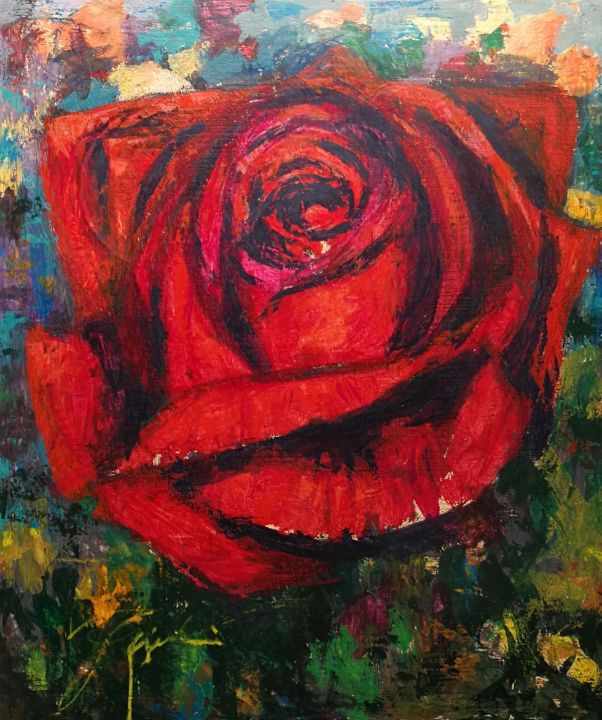The painting prominently features an ornate red rose blossom, rendered in a watercolor or impressionist style that showcases the intricate details of its petals and inner structure. The rose dominates the image, with no visible stem or thorns, and appears deep red with accents of black and pink that enhance its depth and texture. Surrounding the rose, the background is a mesmerizing blend of multicolored watercolors. At the top, hues of blue and orange are most prominent, complemented by splotches of gray. As the composition extends downward, the colors transition to shades of green, yellow, orange, and flecks of purple, creating an impression of a lush, garden-like setting. The overall effect is one of vibrant, swirling colors that suggest an abstract representation of the rose in a natural environment. There is no visible signature on the painting.